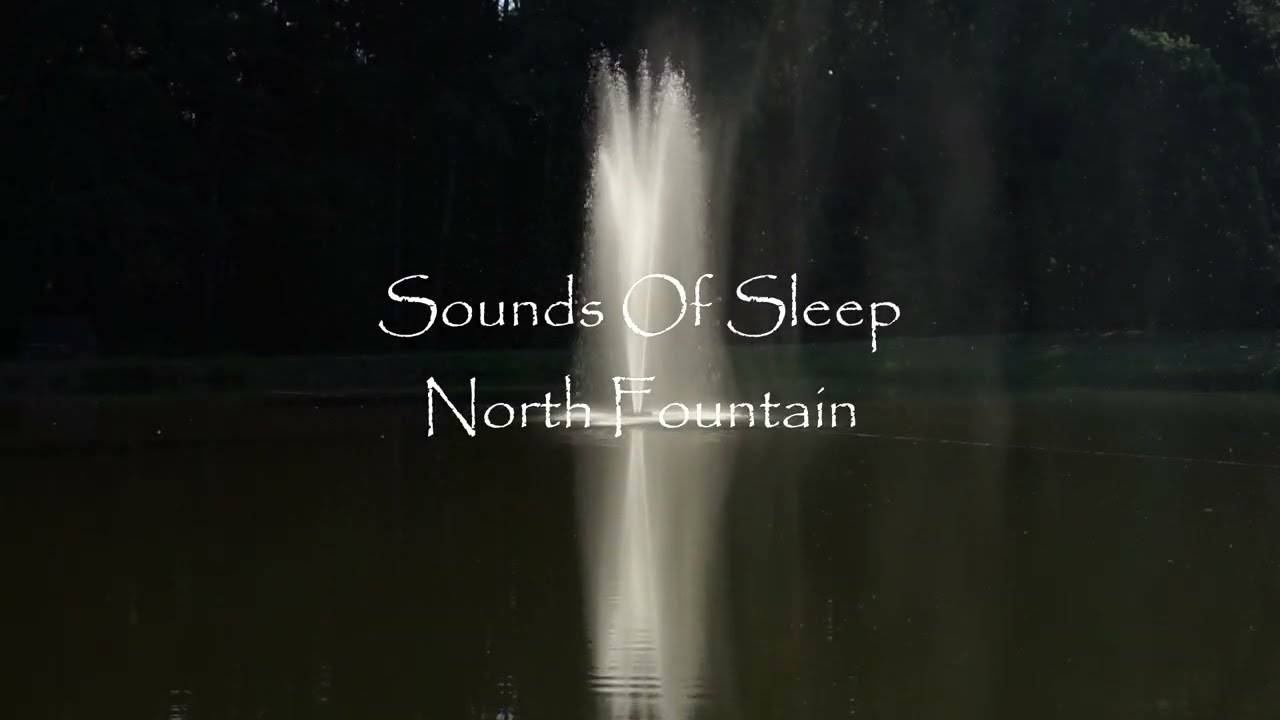The image features a dark, long, rectangular shape with a shadowy scene that is difficult to discern. Central to the image is a grey and white smudge, giving a vague impression of people, trees, and water, possibly a lake or pond. Dominating the top middle is a fountain, its white spray stark against the darkened background. The bottom portion of the image extends into the lake or pond, showing a reflection of the fountain. Across the middle, in bold white text with a unique font that looks almost printed, are the words "Sounds of Sleep," with "Sounds" partially in uppercase. Below this, the text reads "North Fountain." The entire backdrop is enveloped in near-black shadows, with indistinct hints of bushes or trees in the upper right corner, contributing to the mysterious ambiance.